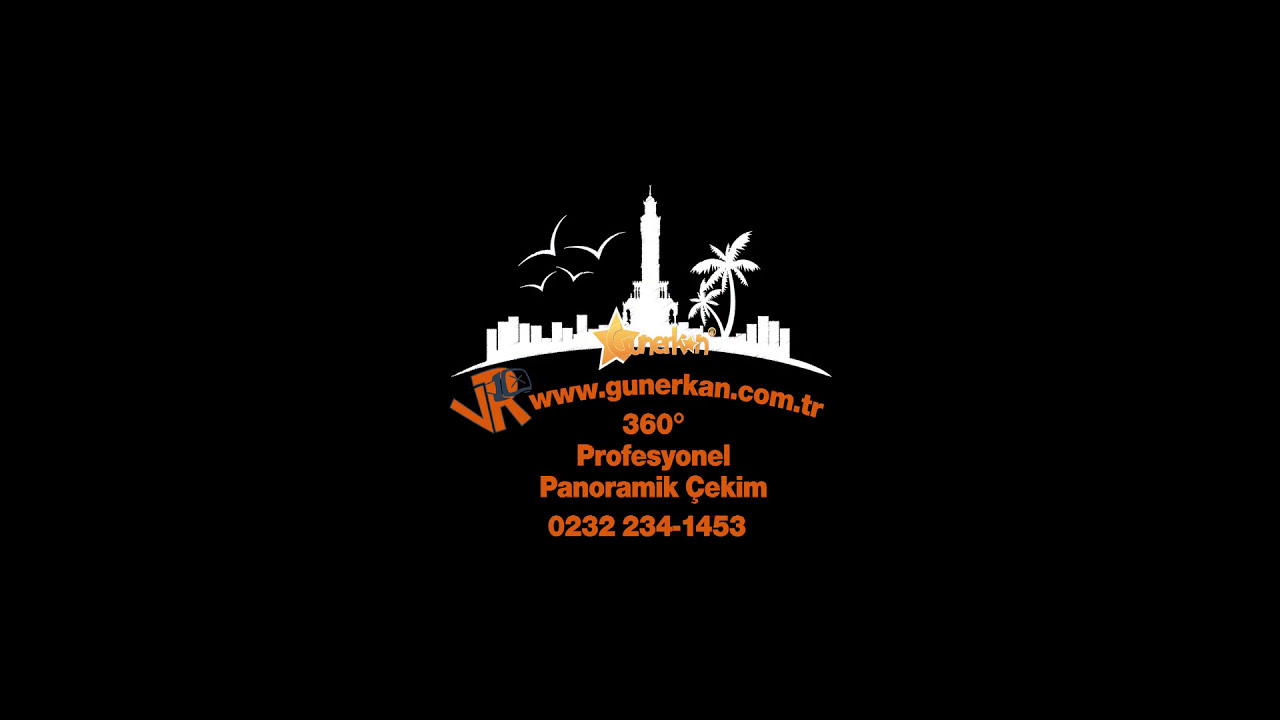Against a solid black background, this scene features a white silhouette logo at its center depicting a tropical cityscape. A prominent tower rises in the middle, flanked by palm trees on the right and smaller buildings on either side. In the sky above, birds—represented as simple ‘V’ shapes—fly past. Below the cityscape is a gold star with partially obscured text that appears to read "Gunerkan." Surrounding the logo in an arc are orange letters stating "www.gunerkan.com.tr, 360 degree, professional panoramic secum," accompanied by the phone number 0232-234-1453. This seems to be an advertisement for a company offering some type of 360-degree panoramic service.